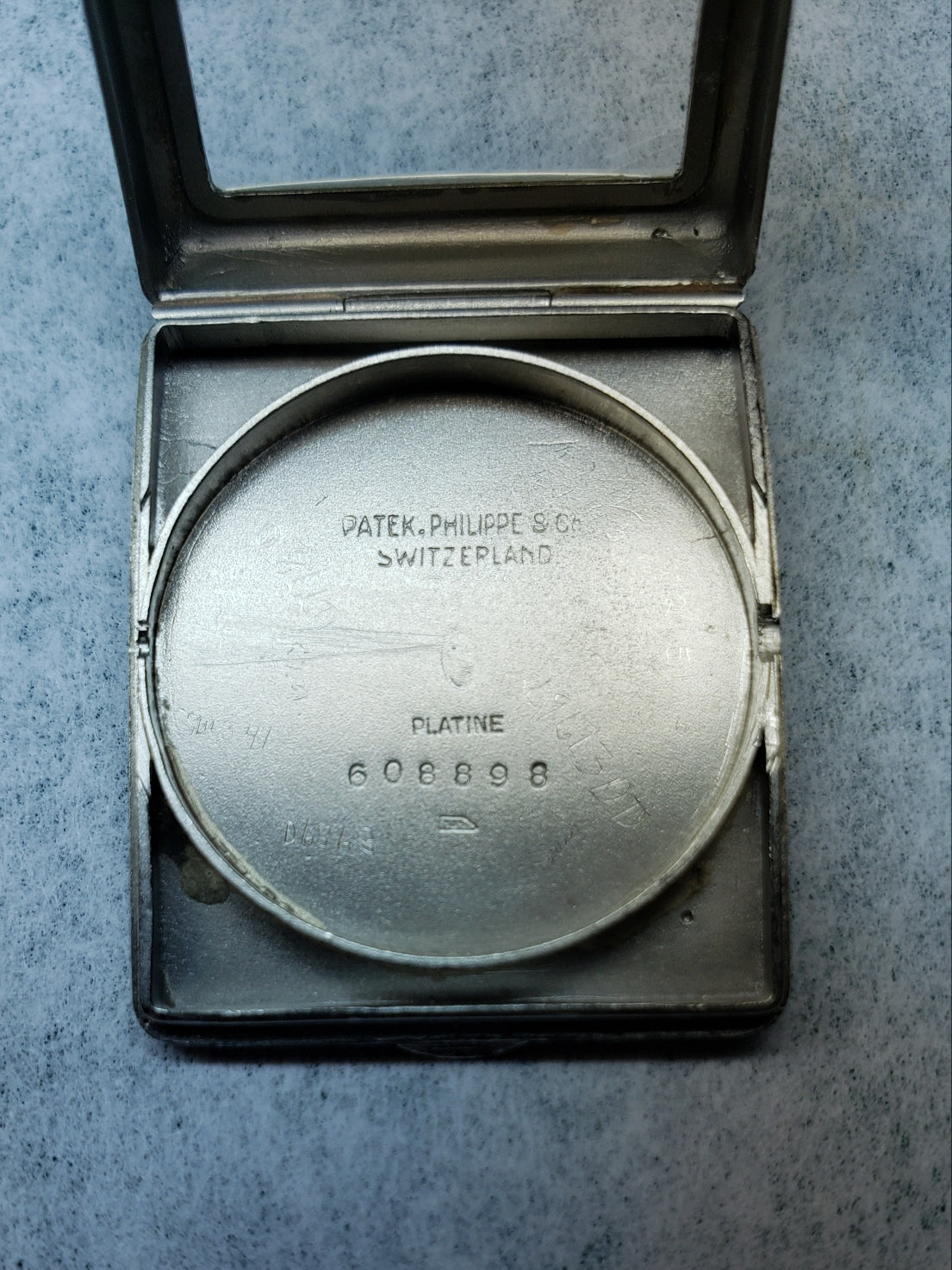This image features a centered, open rectangular metal case with a clear, hinged lid revealing its contents. The background consists of a subtly textured, criss-crossed pattern of blue and white lines, resembling a stone or similar surface. The case itself appears silver, though it has a black edge that frames it. 

Inside the case, occupying approximately 75% of the image's central space, is a silver oval plate with a raised border. The plate is engraved with the text "Patek Philippe SC" at the top center, "Switzerland" directly beneath it, followed by "Platine" which is the Swiss term for platinum, and the number "608898" below that. There might be additional, less prominent numbers or stamps indicating the composition or authenticity of the item.

The oval plate and its detailed engravings suggest it may be an important piece for a high-end product, possibly related to Swiss watch craftsmanship, such as a placement piece or part of a watch mechanism. The precise materials and craftsmanship, along with the meticulous engraving, indicate a luxurious and significant item showcased on a sophisticatedly textured background.